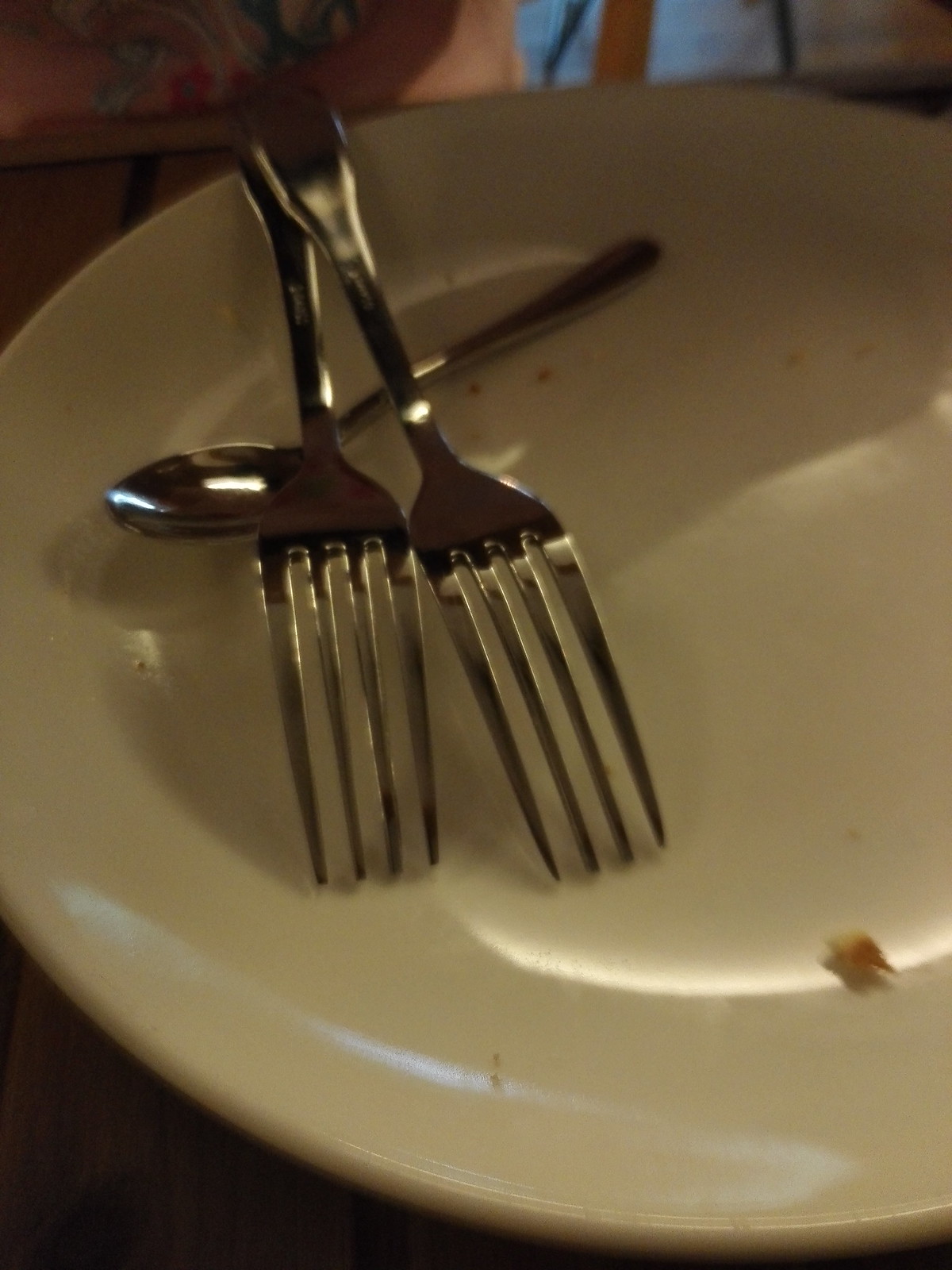In this image, there is a large white plate with brown crumbs scattered across its surface, indicating remnants of a recently finished meal. Positioned at the left side of the plate are two shiny, chrome-like silver forks standing upright with their ends attached to the base of the plate and the forward parts inside. Beneath these forks is a silver spoon, positioned upright and facing left. All three utensils gleam strikingly under the light. The plate rests on what appears to be a dark wooden table. In the background, there is a pink pillow with a floral design and a glimpse of a person wearing a blue shirt, along with what looks like a brown cabinet, adding to the homely setting of the scene.